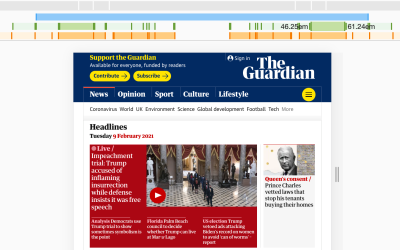This image appears to be a reduced-size screenshot, likely from a website, making finer details difficult to render correctly. At the top, there is a thin gray line followed by a blue line, beneath which a series of green lines is interspersed with darker green bars. On the right-hand side, black text displays measurements: "46.25 and 61.24 cm". Below this, an orange line mimics the pattern of the green line, composed of orange sections separated by darker orange vertical lines.

A dark blue banner marks the bottom of the section, where the upper left corner contains a yellow text that reads "Support the Guardian," while the upper right corner features "The Guardian" logo in white. Just above the logo, white text states "Sign In." On the left, there are two oval buttons labeled "Contribute" and "Subscribe" in black text. Beneath these buttons is a thin orange line, and horizontally along the top left, white labels read "News, Opinion, Sport, Culture, and Lifestyle." The far-right corner has a yellow circle with three horizontal black lines indicating a menu icon.

Below the blue section, a white background hosts a line of black text that is difficult to decipher. In bold black text below this, it says "Headlines, Tuesday," and appears to indicate the date "9 February 2023" in red, although it’s blurry. Below this date, a red rectangle with white text contains a video thumbnail in its upper right corner. The thumbnail seems to depict a formal event, possibly in a museum or ballroom, filled with statues and people in suits. In the top left corner of the red rectangle, partially legible text begins with "Live" and mentions Trump, although the full context is unclear. The upper right corner holds a small black and white image of Prince Charles, accompanied by his name in black and an unreadable red headline below it.